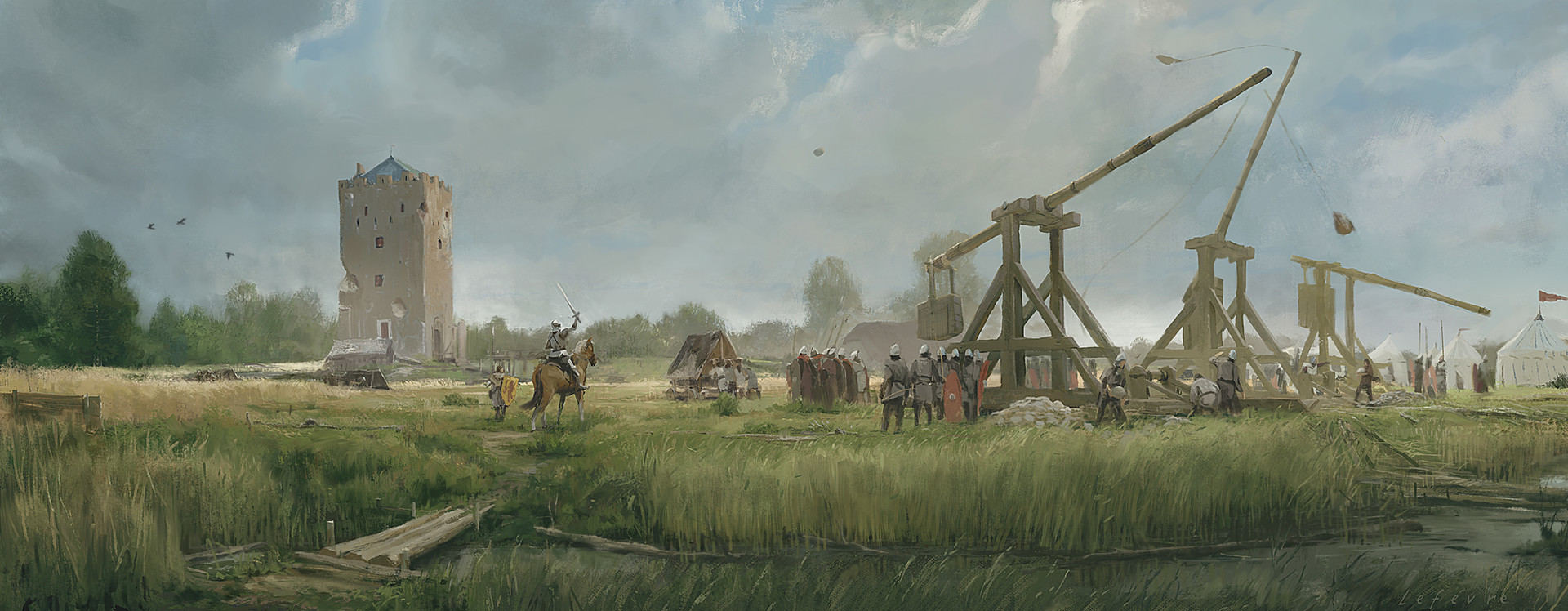The image depicts a painting of a historical scene that evokes a sense of the 1800s, potentially from a Civil War time period. The foreground is adorned with long, green grasses, leading the eye to an array of figures and machinery in the mid-ground. The machinery appears to be large, wooden catapults poised as if ready to launch rocks or boulders. Scattered around these devices are soldiers dressed in gray with red accents, some wearing helmets. Near them are brown horses and a few camping tents, adding to the military atmosphere. Among the soldiers, a figure resembling a general holds a sword aloft, suggesting readiness for an impending charge. To the left, there's an old-fashioned building or tent structure, while in the background, a light brown brick tower with windows stands tall against a light blue sky dotted with white clouds. The scene is enveloped in a dim light, with dirt and clouds adding a muted, almost eerie quality to the overall composition. The landscape is also dotted with green trees, enhancing the painting’s depth and historical ambiance.